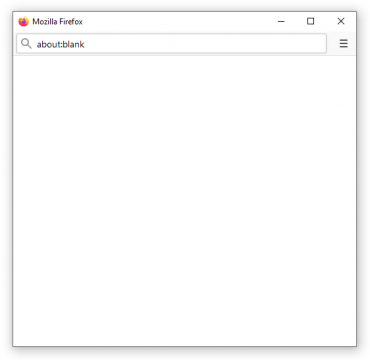The image depicts a blank Mozilla Firefox browser page. The page is encapsulated within a square or rectangular box that features a subtle gray outline and a light gray shadow, enhancing its visual effect. In the upper left corner inside the box is the Mozilla Firefox logo. This logo consists of a blue circle encircled by an orange border, which transitions from an orangish-red hue at the bottom left to a yellowish-orange hue at the upper right. 

To the right of the logo, the text "Mozilla Firefox" is prominently displayed. At the far right of the top border, there are the typical web navigation icons: a horizontal line for minimizing the window, a square for maximizing or creating a new page, and an 'X' for closing the window.

Below these elements, a search bar is situated. This search bar has a light gray outline with rounded corners, and on its far left, there is a gray magnifying glass icon followed by the text "about:blank." The majority of the search bar is blank white space extending to its right edge. Adjacent to the right end of the search bar is a menu icon represented by three horizontal lines in a lighter gray section.

The rest of the browser's interior is predominantly plain white space, providing a clean and uncluttered look.